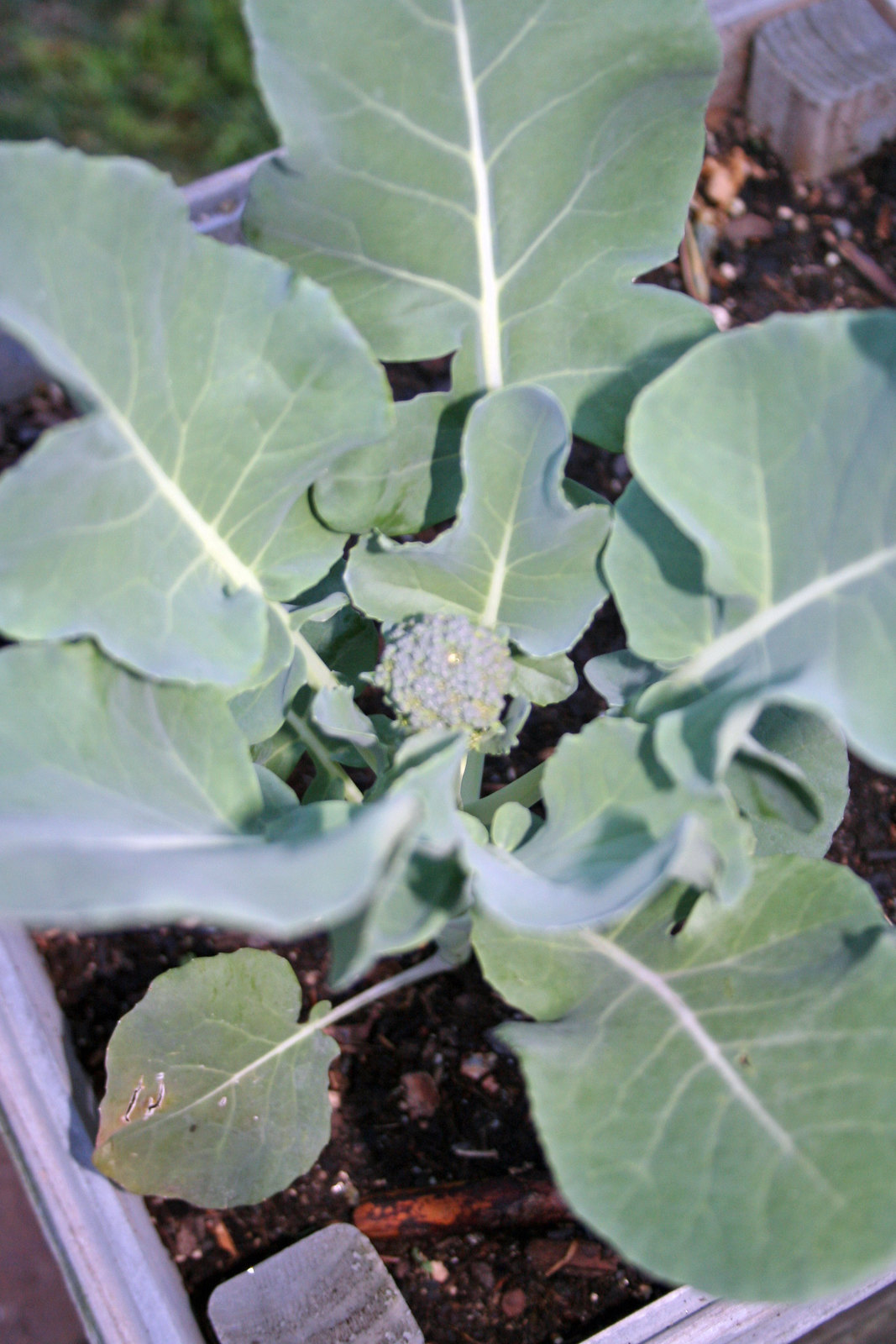The image is a detailed, top-down color photograph of a young broccoli plant growing in a square, wooden raised garden bed. The rich, dark brown soil, interspersed with organic matter and compost, fills the planter, which is bordered by grayish wood. In the center of the image, the broccoli plant features large, well-developed, broad green leaves with prominent white veins that give them a slightly powdery appearance. These leaves fan out from a tiny, central broccoli floret, no larger than a quarter, which is beginning to form. The edges of the wooden container are visible around the plant, with stakes holding the corners together. In the background, on a lower plane, grass or lawn is visible, providing contrast to the elevated garden bed. Small pieces of wood can also be seen in the soil, possibly used to support the plant's stems.